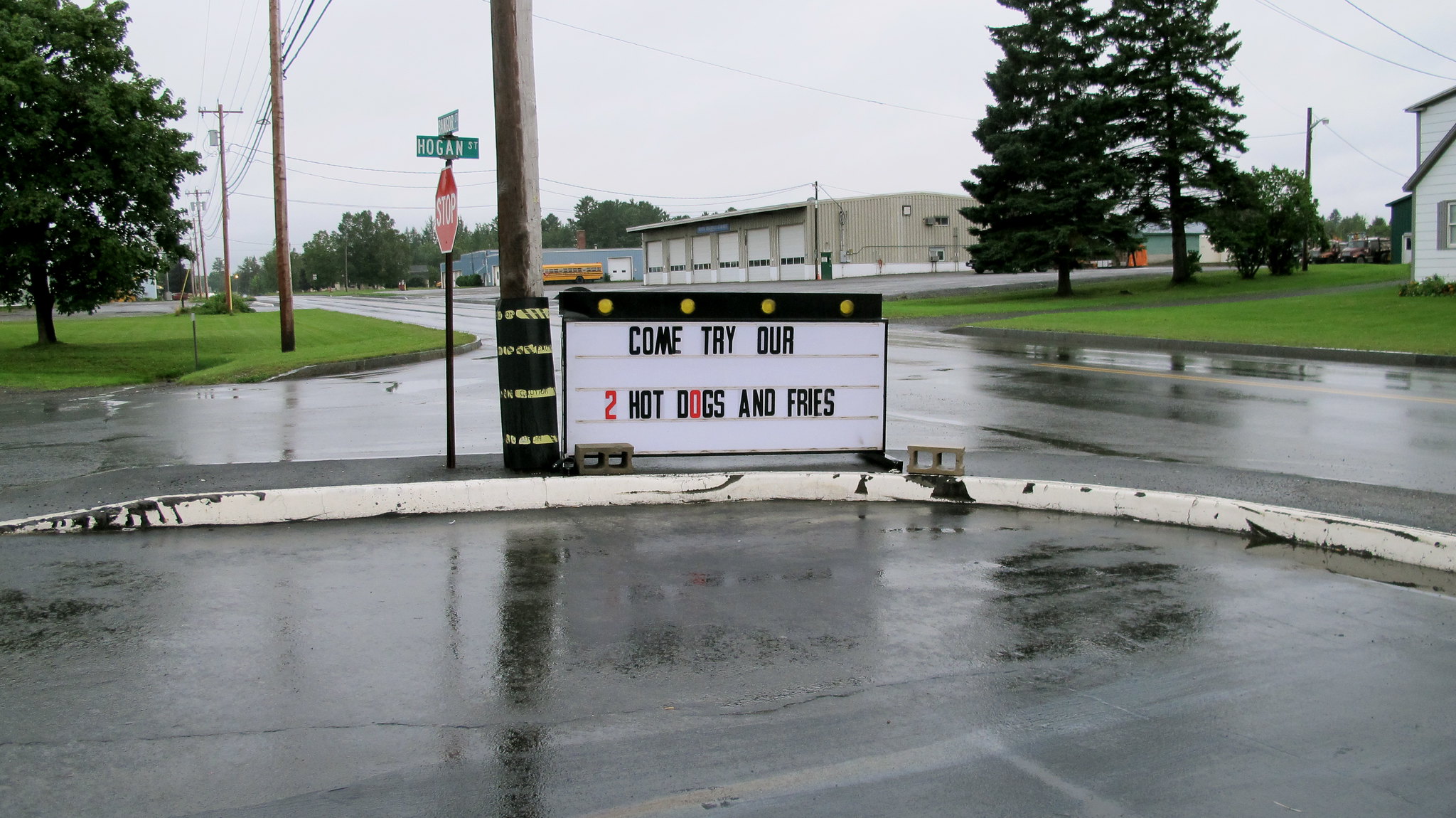Captured in the midst of a rainy day, this photograph showcases a glistening street corner with wet pavement and small puddles scattered about. To the left, an urban intersection is marked by a prominent stop sign alongside street name signs, one of which reads "Hogan." Just behind the stop sign stands a power pole, a line of which stretches down the left side of the street. To the right of the intersection, a large white sign with black letters invites passersby to "Come try our two hot dogs and fries." This enticement is positioned toward the photographer’s vantage point at the corner. In the scene’s backdrop, a street winds from right to left, bordered by various buildings and a patch of grass. Tall trees rise majestically on the far side of the street, adding a touch of nature to the urban setting while hinting at the expansive line of power poles that continue into the distance.